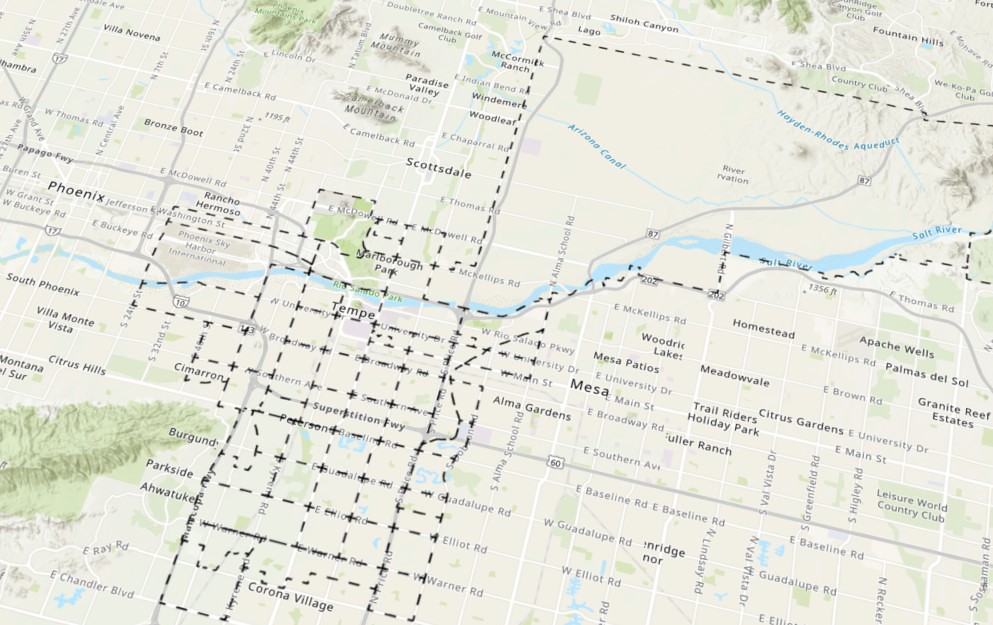The image depicts a detailed road map of Arizona, showcasing an extensive network of cities and roads, laid out in a clear, grid-like pattern. Prominent cities are labeled, including Phoenix on the far left, Scottsdale near the center top, Tempe in the middle, and Mesa slightly to the right. Various smaller towns are also marked on the map. Topographical features are prominently displayed, highlighting mountains, hills, and rivers. A notable green mountain with visible elevation is located on the left-hand side of the map. The Salt River runs through the center, accompanied by other smaller waterways. Additionally, there are checked lines following certain roads, possibly delineating regions or townships, which traverse up the map before turning sharply to the right.